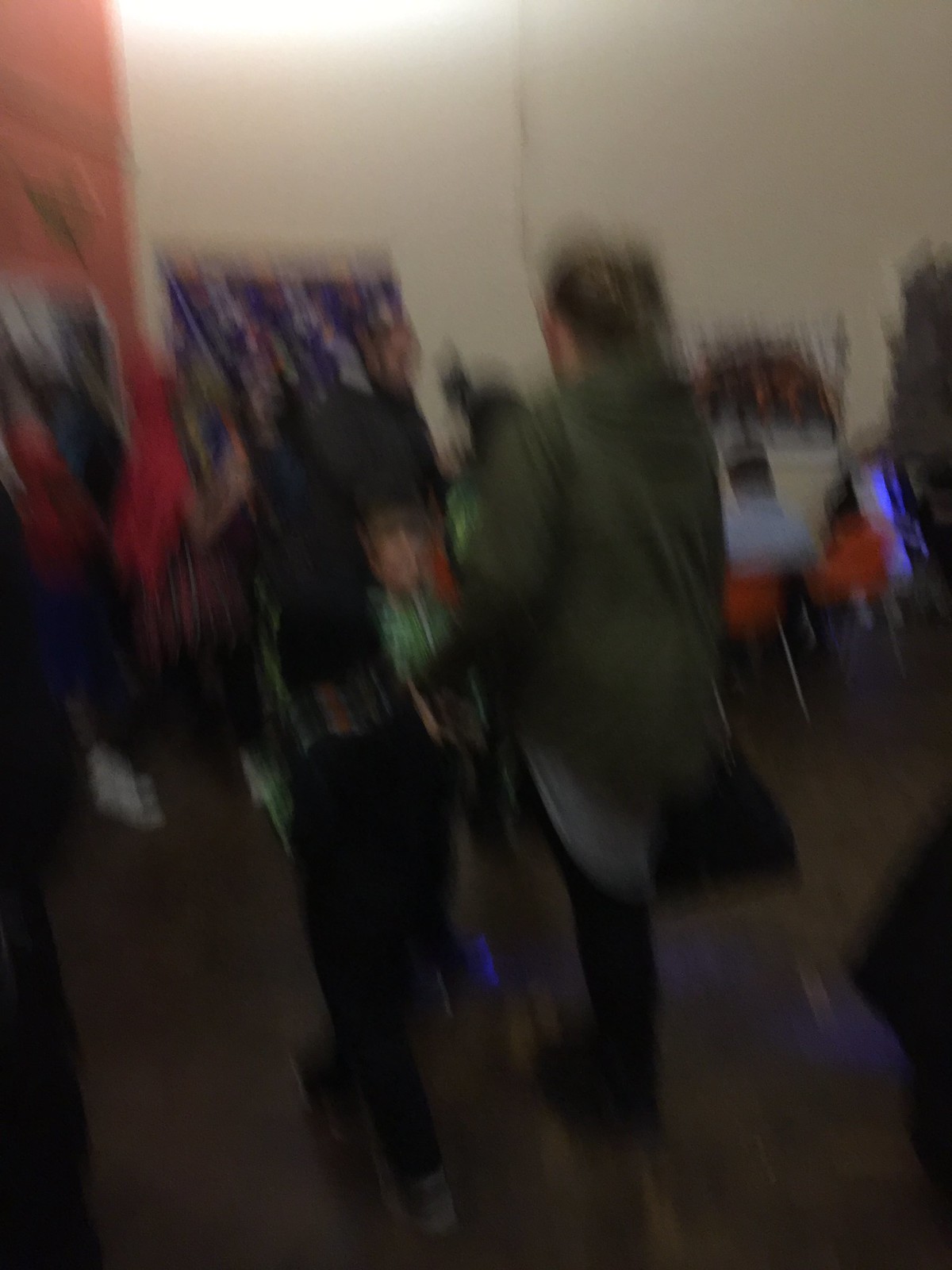This is a highly blurred, diagonally skewed portrait-style photograph, likely caused by the photographer's movement or camera shake while taking the picture. The image seems to depict the interior of a bustling building with white walls and ceiling lights. A line of red chairs is positioned against a wall adorned with two posters. Seated in these chairs, which are possibly set up at computer stations given the monitor lights, are a few individuals who are just barely distinguishable due to the motion blur.

In the foreground, the main subjects are a woman with her back to the camera and her child, who might be facing the lens, although the heavy blur makes it difficult to confirm their orientation or expressions clearly. Additional people can be seen scattered throughout the scene, contributing to the sense of activity, though their actions and identities are obscured by the image's lack of focus.